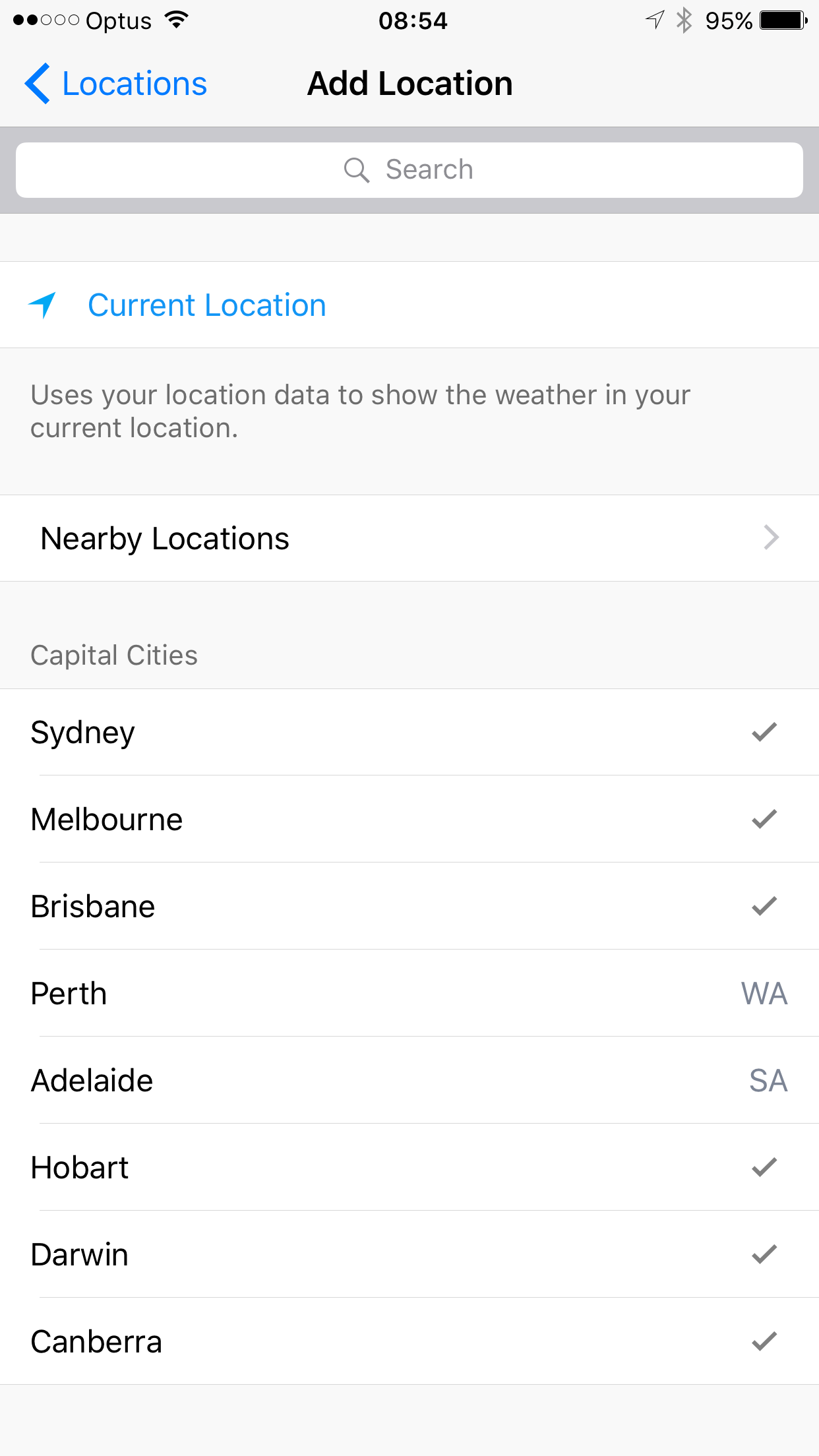Screenshot of a mobile device displaying a weather application interface:

At the top of the screenshot, you can see the mobile device's status bar. On the top left, five connectivity dots are displayed, with two of them blacked out. To the right of the dots, the network name "Optus" is shown, followed by a Wi-Fi icon. In the center, the current time is displayed as 08:54. To the right, there are icons for location services, Bluetooth, and the battery level which is at 95%.

Below the status bar, the weather application interface begins. The top of the page features the title "Add Location," with a blue button labeled "Locations" to its left and a left-pointing arrow next to the button. Directly beneath the title is a search bar.

Continuing downward, there is a prominent blue button labeled "Current Location," featuring a location symbol with an arrow pointing upwards and to the right. Below this button, there's an explanatory text: "Use your current location data to show the weather in your current location."

Following the text, there are several toggle options. The first toggle reads "Nearby Locations." The next section is titled "Capital Cities," listing the following cities: Sydney, Melbourne, Brisbane, Perth (marked with "WA"), Adelaide (marked with "SA"), Hobart, Darwin, and Canberra. All cities have a check mark next to them except for Perth and Adelaide.

The overall design of the app interface reflects a minimalistic style characteristic of iOS devices, featuring signature white and gray backgrounds with blue accents.